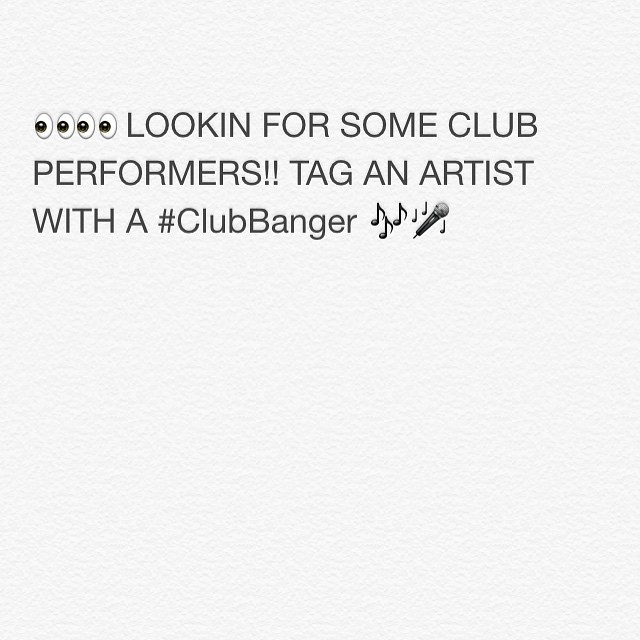The image is a textured, white, paper-like background with a social media post in a sans serif, dark gray font. The text is left-aligned near the top, surrounded by a generous amount of white space. The content begins with four eyeball emojis looking to the left, followed by an all-caps statement: "LOOKING FOR SOME CLUB PERFORMERS!! TAG AN ARTIST WITH A #ClubBanger." After this call-to-action, there are musical note emojis and a line art symbol of a microphone with additional music notes, angled up towards the top right. The design evokes a tweet or social media post, with the typography and positioning giving it a clean, minimalist look.